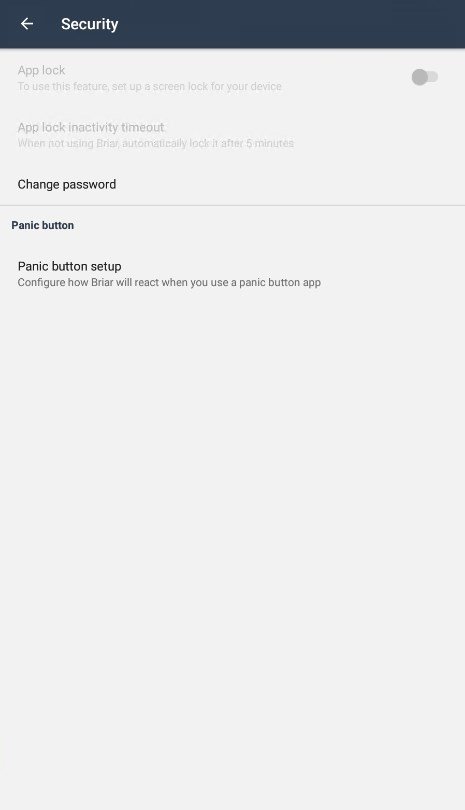This image appears to be a screenshot taken from a smartphone within the settings menu, specifically focusing on security settings. At the top of the image, there is a long blue title bar with a white arrow pointing right in the left corner, next to the text "Security" in white font. Below this, there are some faded options: 

- "App Lock": It prompts the user to set up a screen lock to use this feature.
- A toggle switch for activating the App Lock is present but currently appears to be off. This whole area is grayed out, making it difficult to read the text.
- "App Lock and Activity Timeout" followed by text that suggests configuration for when the device is not in use, mentioning a 5-minute timeout.

Further down, "Change Password" is prominently displayed in bold black font with a thin line spanning the width of the image beneath it. Below this, there is a "Panic Button" section, in smaller font, which includes options for setting up the panic button. This section explains that it allows the user to configure how the app "Briar" will respond when a panic button app is used.